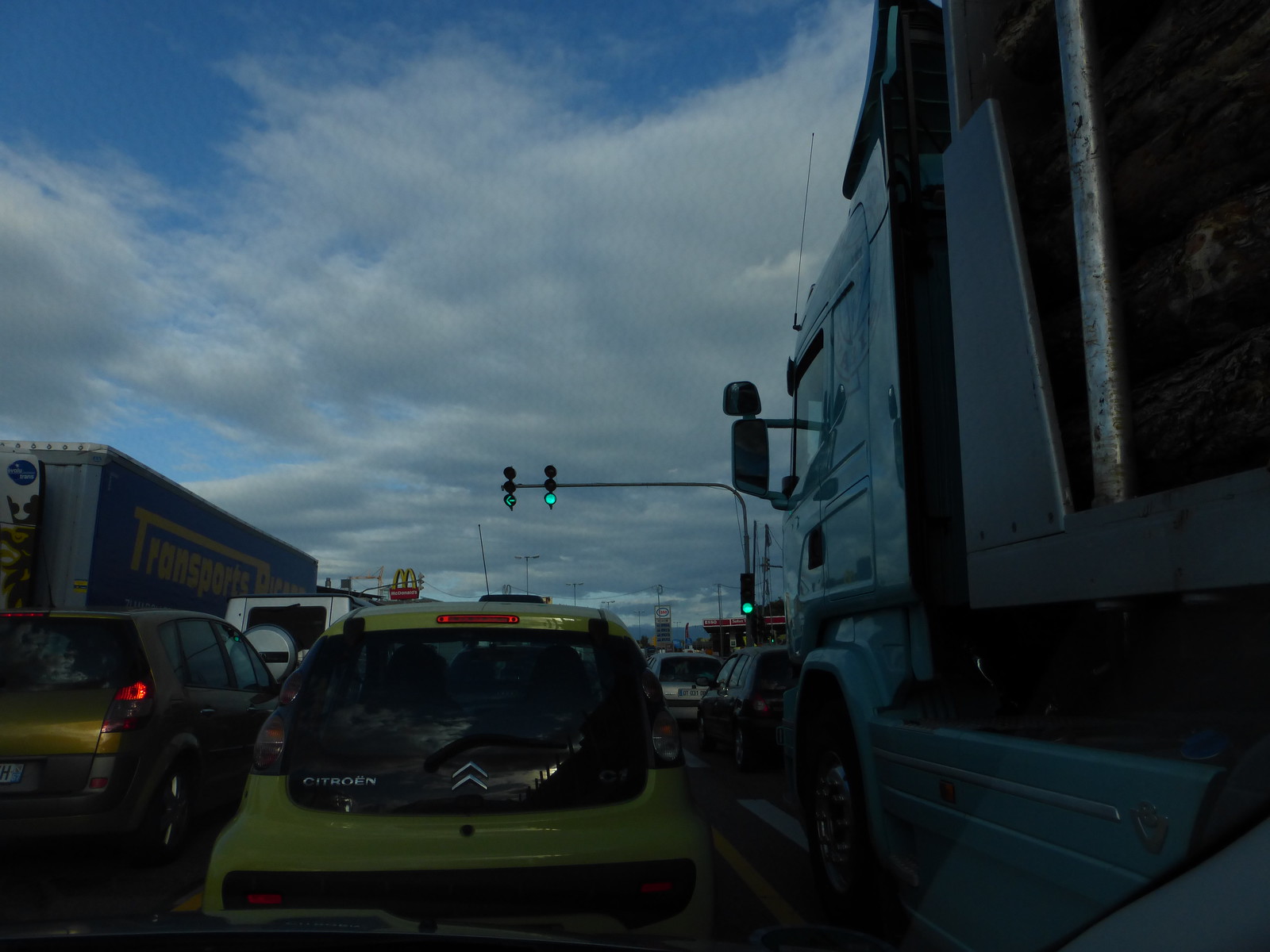In this dimly lit exterior shot, either at dusk or dawn, we observe a busy highway section with traffic stopped at a green light, preparing to move. The sky is a gradient of blue with sheets of whitish-gray clouds. Through a windshield, we see multiple vehicles: directly ahead is a lime green sedan, to the right is a dark blue semi-truck with yellow writing that partially reads "transports." To the left, there is a gold SUV-like vehicle with a dark-tinted rear window and in front of it, a silver or white Jeep-like car, also with a dark back window and a spare tire mounted in the back. In another lane, there's a dark blue box truck. Hanging overhead on a silver pole are traffic lights: one with a green arrow pointing left and another with a solid green light. Additional green lights are seen partway up the pole on the right. In the background, identifiable structures include the top of a McDonald's sign and other buildings, possibly including a gas station marked by red and white signage.